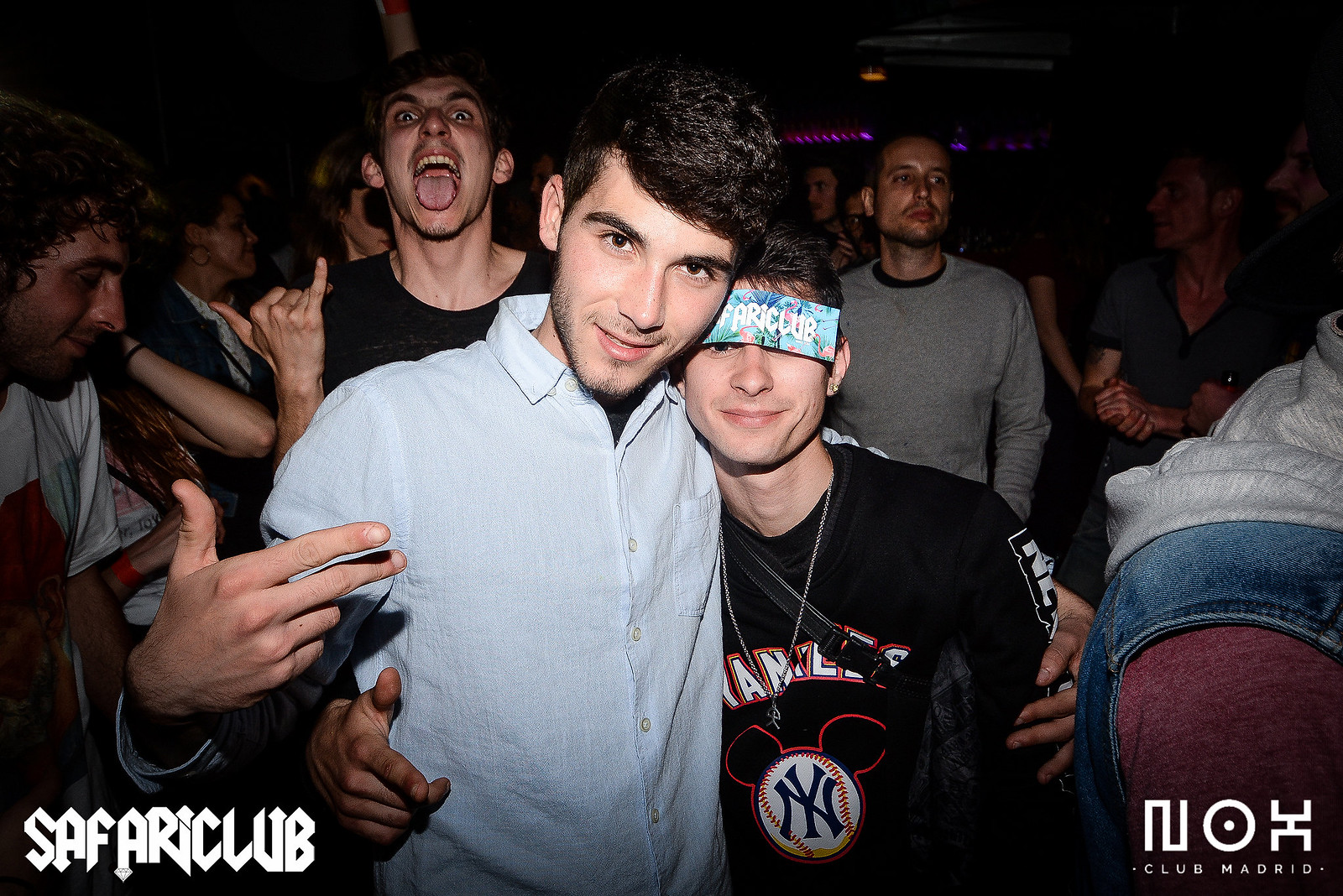This lively photograph captures a dynamic club party atmosphere, prominently showcasing the energetic ambiance of Safari Club and Club Madrid, as indicated by the text in the bottom left and right corners. In the foreground, two young men take center stage: one on the left wears a light blue dress shirt, smiling warmly at the camera while extending his right hand out and wrapping his left arm around his friend. The friend, adorned in a black long-sleeved New York Yankees shirt with a Mickey Mouse symbol, has a ticket pasted to his forehead and is also beaming at the camera. Adding to the festive spirit, a third guy stands just behind them, mouth wide open in a scream, tongue sticking out, and flashing the rock on sign. The background is filled with a colorful array of party-goers dancing and enjoying the night, all contributing to the vibrant scene that is equally a spontaneous moment and a potential advertisement for Safari Club and Club Madrid. The photograph vividly captures the joy and excitement of a night out at the club in Spain.